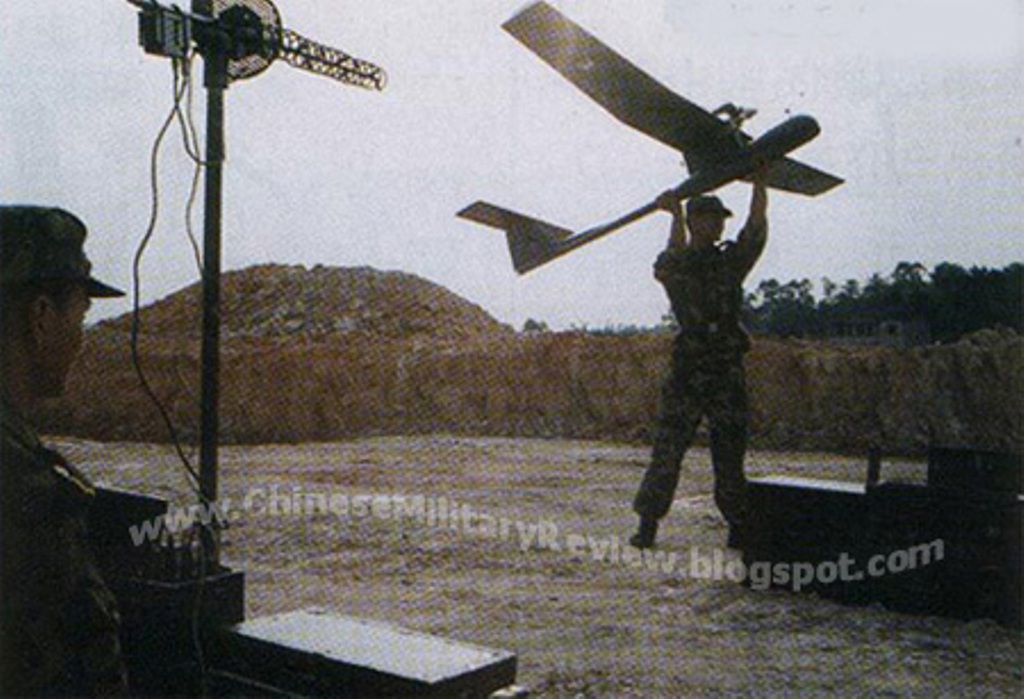This is a grainy, low-resolution color photograph, likely taken with an old camera or scanned from an older print, giving the image a washed-out appearance with a slight reddish-cyan hue. The outdoor scene features a light gray sky, indicating daytime, and a backdrop of hills, trees, and bushes. The central focus is on a field with tan or light green grass. In this setting, two soldiers in military uniforms are captured; the soldier on the right is holding up a small flying drone or model airplane, presumably preparing to launch it. Nearby, the second soldier on the left stands beside some equipment, which includes a piece of machinery and a small antenna. Due to the lighting, both soldiers appear somewhat silhouetted. Faintly overlaying the bottom portion of the image is a watermark text that reads “www.chinesemilitaryreview.blogspot.com.”